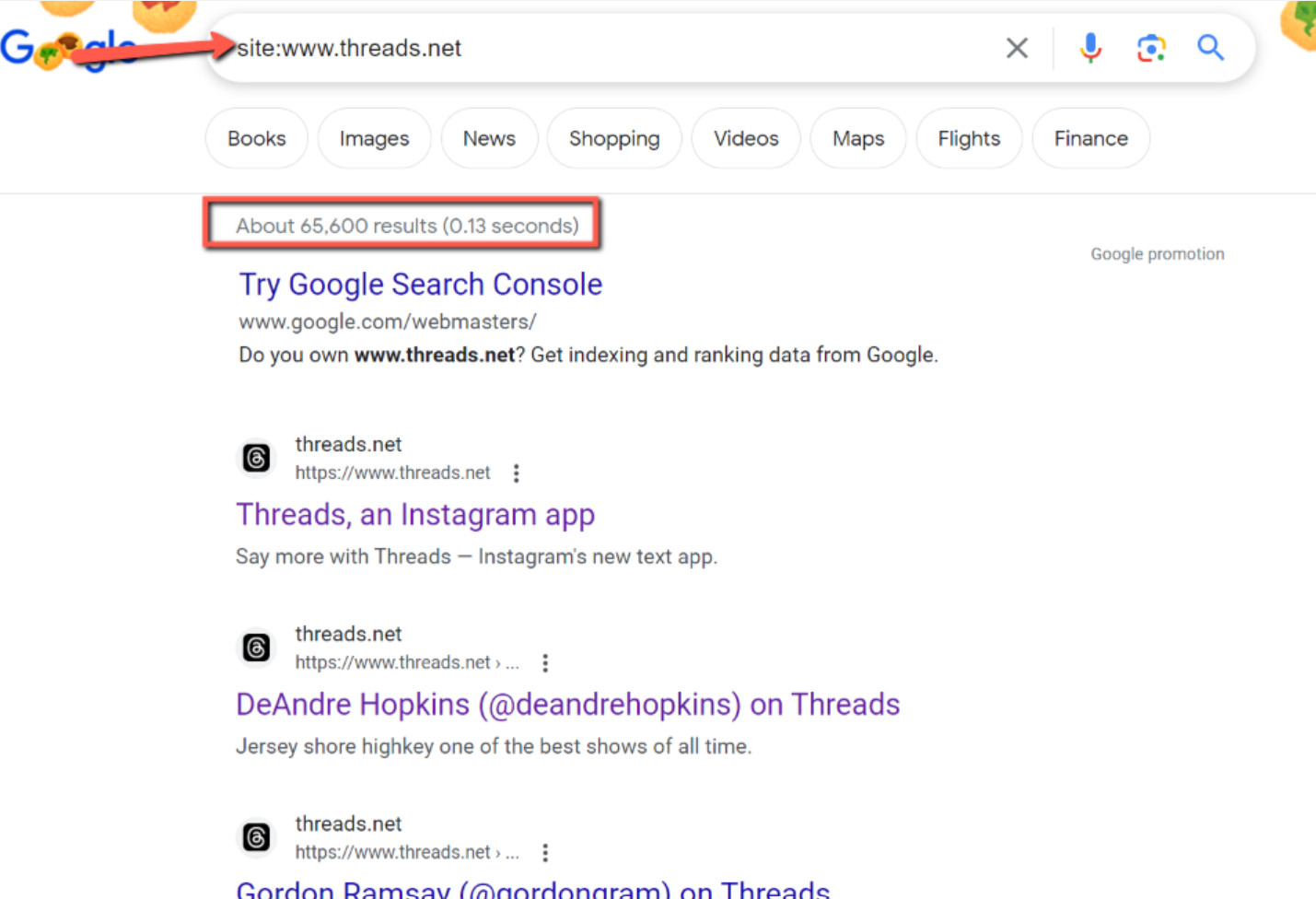In the image, we see a Google search results page. At the top of the page is the search bar displaying the query "site:www.threads.net". Next to the search bar, from left to right, there are icons: a gray 'X' for clearing the search, a microphone icon for voice search, a Google Lens icon for visual search, and a magnifying glass icon, typically for submitting the search query.

Below the search bar, there are eight category tabs in black text: Books, Images, News, Shopping, Videos, Maps, Flights, and Finance. 

Next, a red rectangle highlights a line of text that reads "About 65,600 results."

The search results follow:
1. The first result, highlighted in blue, reads "Try Google Search Console," followed by a description inviting the user to get indexing and ranking data from Google.
2. The second result is for "threads.net," described as "Threads, an Instagram app."
3. The third result is "threads.net DeAndre Hopkins," indicating content related to DeAndre Hopkins with his username in parentheses: (at DeAndre Hopkins on Threads).
4. Within the third result's content, there's a mention of "Jersey Shore" with the phrase, "high key, one of the best shows of all time."
5. The fourth result, partially cut off, references "threads.net" and includes a mention of Gordon Ramsay, indicating his username and that he's on Threads, highlighted in blue.

Throughout the page, small gray text in the top right corner reads "Google promotion." The entire layout stands out against a clean white background.